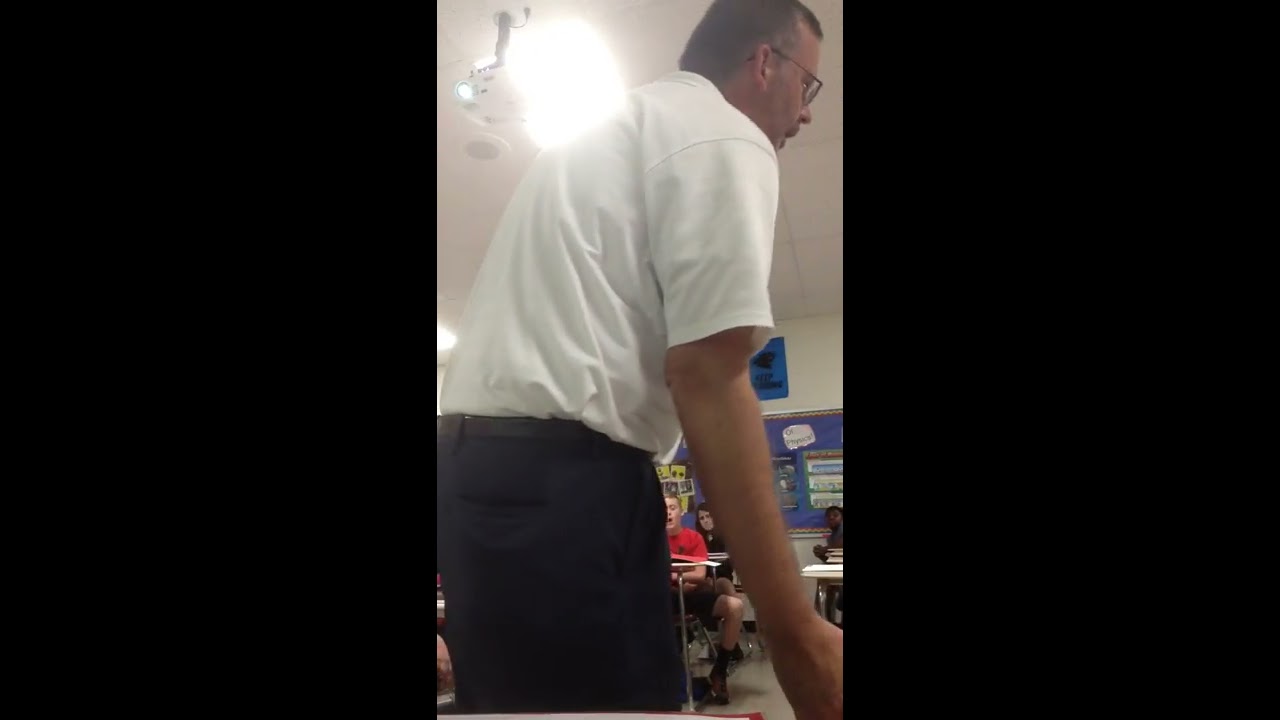The image features a professor standing in a brightly lit classroom, facing towards the right. He is wearing a white collared shirt, black pants, and black glasses, with short dark hair and a light skin complexion. The classroom behind him has white walls and a white tiled ceiling, illuminated by an exceptionally bright fluorescent light directly above his head. Three students are visible at their desks: one in the foreground wearing a red shirt, another behind them in a black shirt, and a third on the far right whose details are unclear. In the background, a bulletin board with a blue background paper displays various ads for events and activities, although the specifics of these ads are indecipherable. Large black bars run vertically down either side of the image, framing the scene. The overall color palette of the image includes various hues such as black, white, red, yellow, green, and blue.